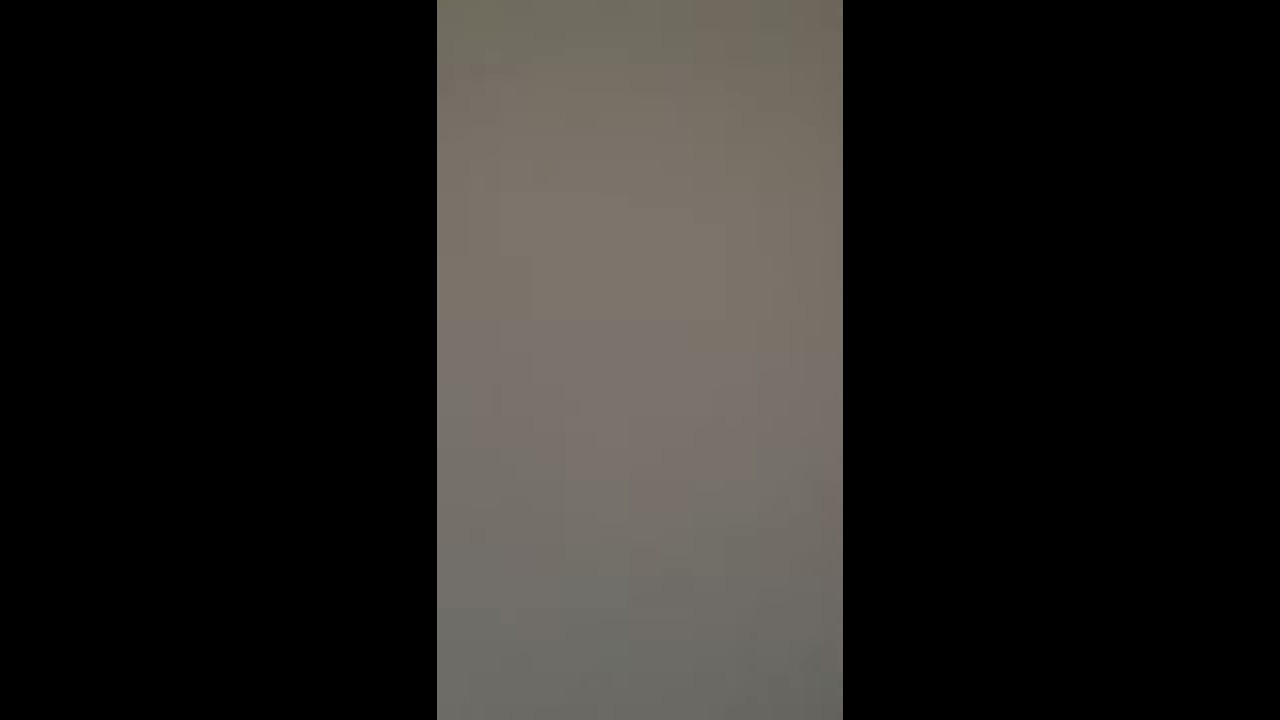The image consists of a horizontally oriented rectangular landscape, divided vertically into three equal sections. Each section is a tall rectangle extending from the top to the bottom of the image. The left and right sections are black, while the center section is a solid, cement-gray panel that occupies approximately two-thirds the width of the black panels flanking it. There is no text or discernible objects within any of the sections, creating a minimalist, abstract appearance. The stark contrast between the black borders and the gray center gives the image a graphic design or potentially a flag-like quality. The uniform height of all three sections enhances the symmetry, while the grayscale color scheme further emphasizes the simplicity and balance of the composition.